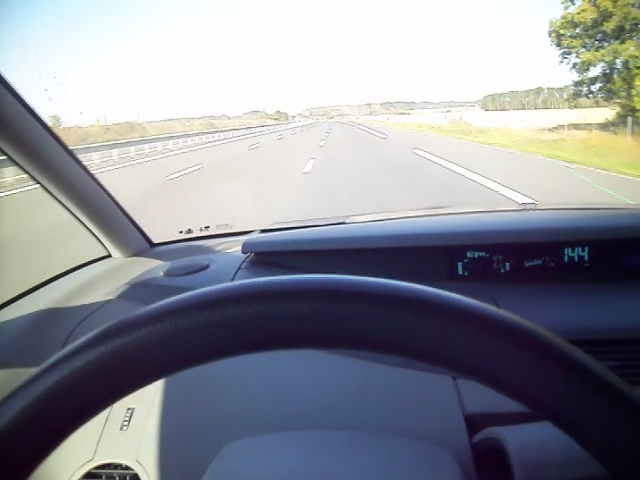This detailed image appears to be a real photograph, capturing the view from the driver's seat of a vehicle traveling on a three-lane highway with a shoulder on the right. The composition features the top crescent of the black steering wheel visible in the bottom left corner, with a grey dashboard showing the number "144" on the right-hand side of the dash, indicating the speed. The dark grey or black interior contrasts with the bright white sky, which also shows hints of blue in the top left corner. The scene outside the windshield includes a metal barrier with white posts on the left side of the road, and a small grassy patch with a green tree prominently visible in the top right corner. The pavement is light grey with white road markings that alternate between dotted and solid lines. In the background, the scene fades into a blur of hills and possibly a body of water, giving the impression of a peaceful highway drive.